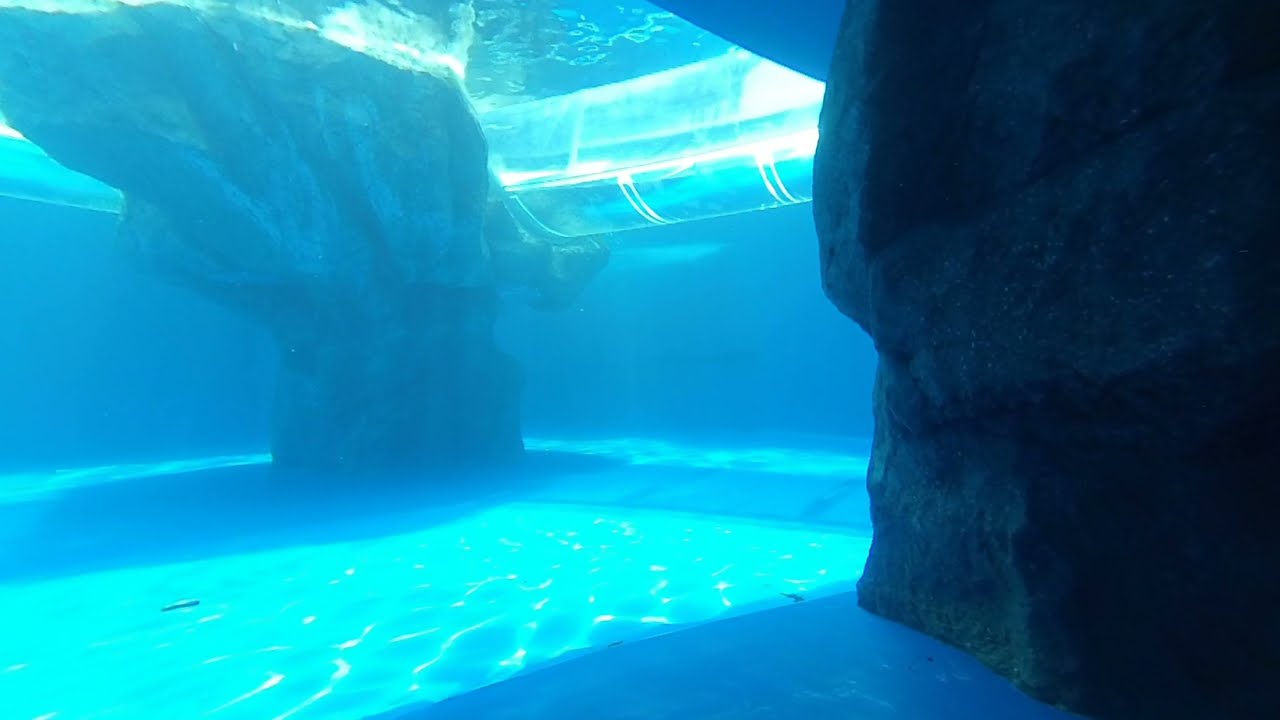This photo captures a serene underwater scene inside a large, man-made aquarium bathed in blue hues with light filtering down from above. Dominating the scene are two rocky, man-made structures resembling stone pillars; one positioned on the far right and the other on the far left of the image. These pillars partially emerge from the smooth, artificial floor that lacks the typical sand and rocks of a natural undersea environment. Suspended between the pillars is a brightly lit, clear tube designed as a pathway, potentially for people to move through. The scene is devoid of any aquatic life or humans, emphasizing the emptiness of the vast tank. The overhead light enhances the reflective, rippling surface of the water, adding to the tranquil, yet distinctly artificial, ambiance of the underwater room.